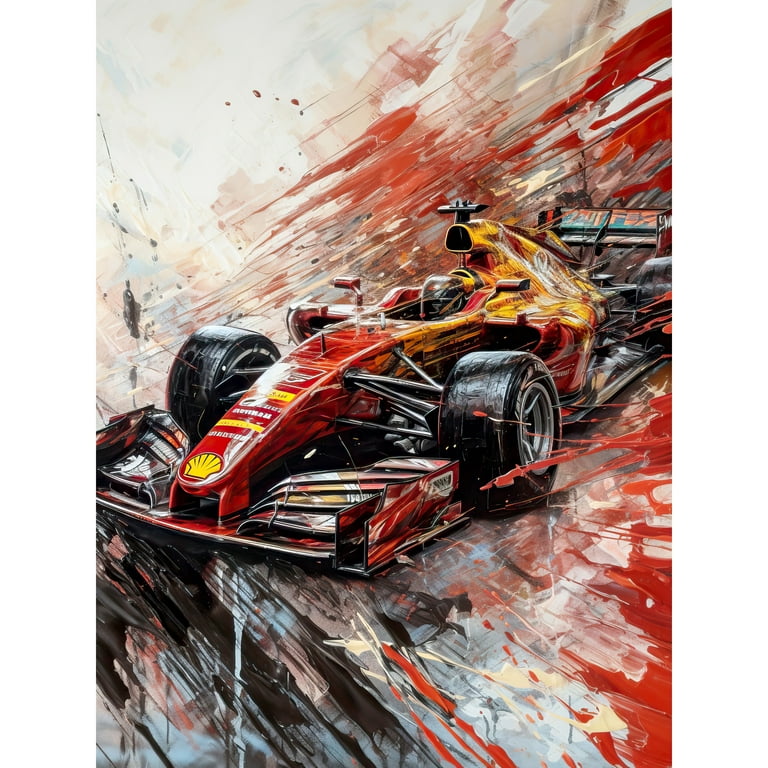This vibrant, oil-painted, color portrait captures the thrilling essence of a speeding Formula One race car, prominently displayed on a stark white canvas. The red car, rendered with meticulous detail, features large, fat black tires and is adorned with a yellow Shell Oil insignia on its front hood. The car is diagonally positioned, with its front facing the lower right corner and rear aimed towards the upper left, conveying a dynamic sense of movement. The rear area, just behind the driver's seat, showcases a blend of yellow and red hues, complemented by a black spoiler.

Artistically applied streaks of red and black paint, along with splashes of blue and orange, radiate from the vehicle, enhancing the visual perception of speed and power. These streaks flow from the left center down to the lower left corner, and from the upper right towards the left center, seamlessly integrating with the car’s motion. The presence of a driver, distinguished by a black helmet, adds to the realism of this energetic portrayal. The composition’s dynamic brush strokes and color contrasts effectively capture the adrenaline-fueled excitement of a high-speed race.